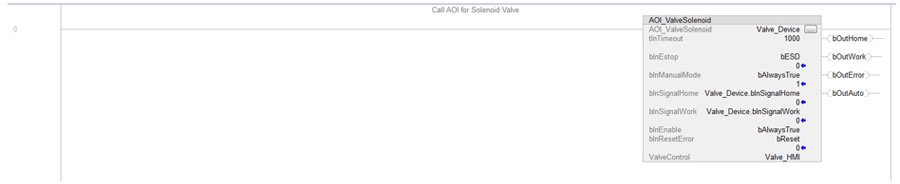The image depicts a detailed schematic with the following elements:

- At the top, there is a very thin gray line positioned about an eighth of the way from the right-hand side. This line extends down, stopping just about a quarter of the way.

- Another gray line runs horizontally across between these vertical lines, intersecting the white area.

- In the center of the white area, there is gray text that reads, "call AOI for S... value."

- More towards the right-hand side, there is a small gray box. The top of this box is darker gray, and it features bold black text that reads, "AIO_value_solian."

- Below this box, on the left side, there's an extensive amount of gray text arranged in approximately seven to eight lines.

- On the right-hand side, there is more black text. The top text reads, "value_device," accompanied by a small white check mark next to it. Below this, it mentions "a thousand" under the device label.

- Additional elements include the text "E ESD" with a word next to it and several blue arrows pointing to the left, aligned with some of the values.

Overall, the image is a complex and technical schematic, challenging to interpret without specialized knowledge.